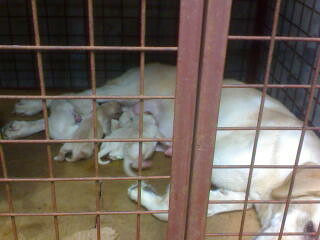This color photograph captures an indoor scene, looking through the wire mesh of a reddish-brown metal dog crate with a windowpane-like square design. The crate features two thicker vertical beams, possibly the edges of the door. Inside, a white and tan Labrador-like mother dog is lying on her left side, with her head towards the lower right of the image, where her right eye, ear, and part of her muzzle are visible. The dog is lying on what appears to be a brown rug or carpet. Nestled against her belly, a group of three to five very young puppies are nursing, their tiny bodies and fur indicating they are just a few days old. This intimate moment highlights the nurturing bond between the mother and her offspring. The dog’s hind legs can be seen towards the left side of the middle of the photo. The crate does not resemble a standard cage and lacks any visible rust, suggesting a well-maintained environment possibly distinct from an animal shelter.